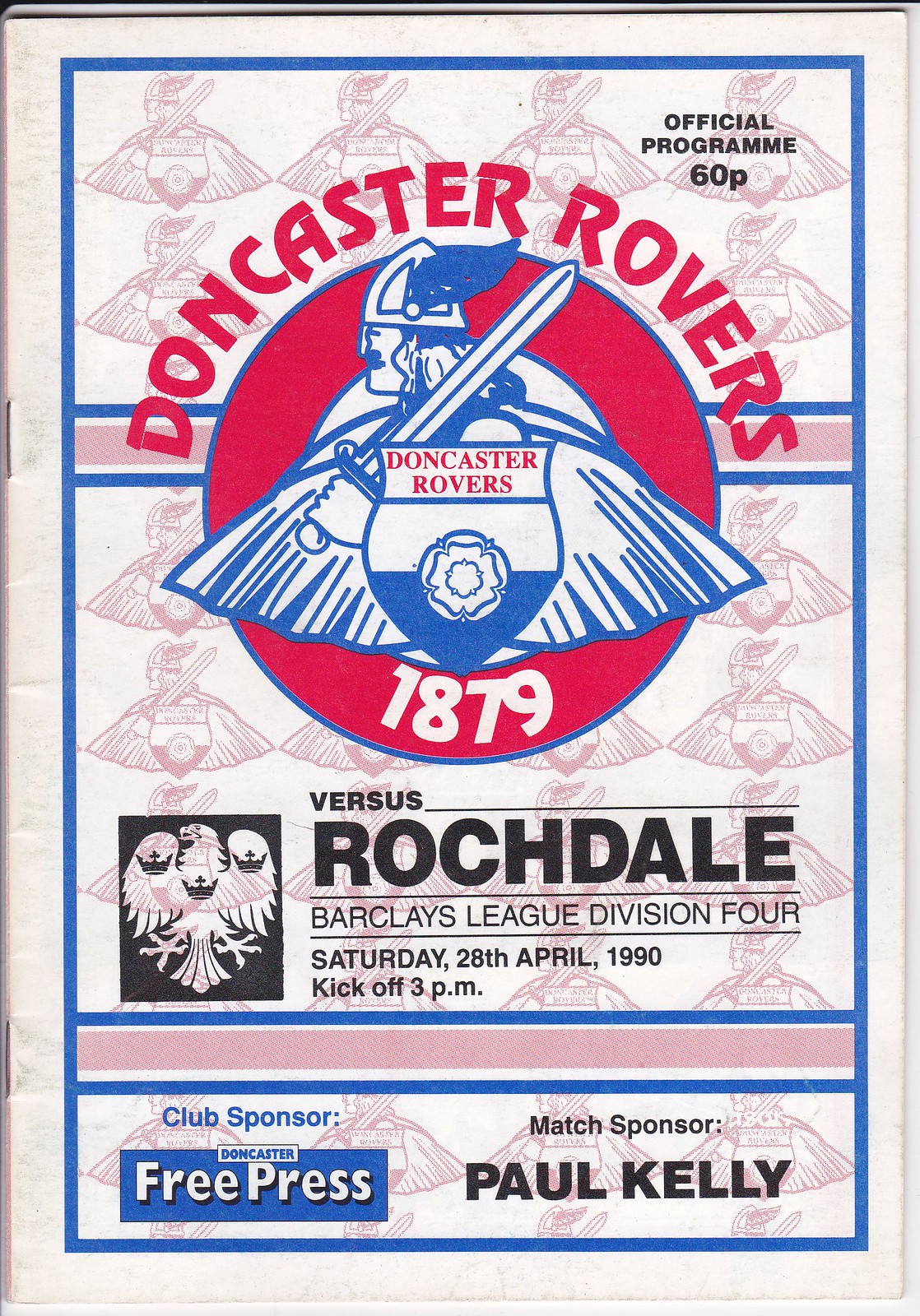The image is a scan of an official program poster for a Doncaster Rovers football match. Featured prominently at the top are the words "Doncaster Rovers" in red font. Below this, there is a large red circle containing multiple detailed elements. Inside the circle is a knight facing left, holding a sword in their left hand, and adorned with a blue and white cape flowing behind them symmetrically. The knight's wide-brimmed hat is also notable. Above the knight is a seal shape; the upper part of the seal is white and the bottom part is blue. Below the seal is a white flower. At the bottom of the red circle, the year "1879" is displayed in white. Outside the circle, on the right side in black letters, it says "Official Program 60p" on a white background. Underneath the circle, in black font, is text that reads "Versus Rochdale, Barclays League Division 4, Saturday, 28th April 1990, kickoff, 3 p.m." In the bottom left corner, there is a blue rectangle labeled "Club Sponsor" and inside it, in white letters, it says "Free Press." To the lower right, it says "Match Sponsor, Paul Kelly" in black font.